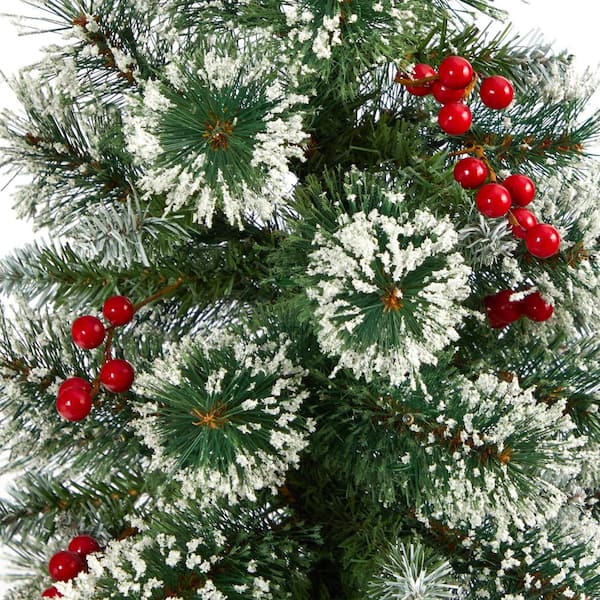This image depicts a close-up of a Christmas tree, likely artificial, given the uniformity and appearance of its features. The tree's branches are adorned with short, pine-like needles, each uniformly tipped with a white, crumbly substance to simulate snow. Scattered throughout the branches are shiny, spherical red berries, which add vibrant splashes of color against the green needles and white "snow." The tree's needles are somewhat bristle-like and identical in length, enhancing the artificial aesthetic. The background is a plain white, providing a stark contrast that highlights the details of the tree. The image captures layers of limbs and clusters of the frosty tips and berries, emphasizing the tree's decorative elements.